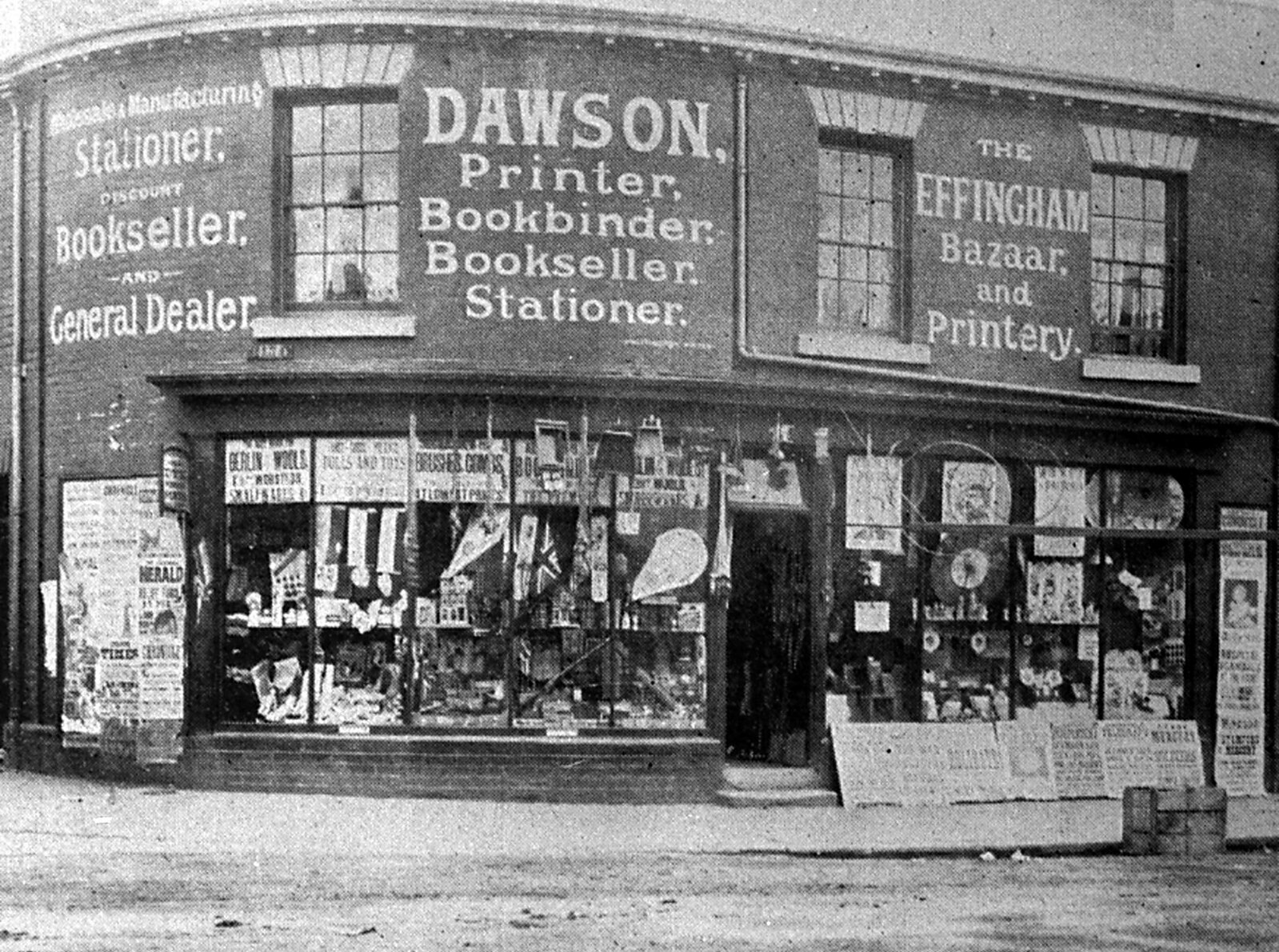The black-and-white vintage photograph showcases a historic two-story brick storefront on a city street, with a slight curve on the left side of the building. The top part of the building is adorned with white-painted signage reading "Dawson, Printer, Bookbinder, Bookseller, Stationer" and "The Effingham Bazaar and Printery." The left side features additional text, "Stationery, Discount Bookseller, and General Dealer." The upper story has two small windows with keystones above them, and the entire facade is covered in various paper signs and newspaper clippings. The bottom floor displays cluttered shop windows filled with more signs and assorted items on shelves, suggesting a bustling but perhaps outdated business environment. The presence of so much paper taped to the windows, along with the painted brick, reinforces the building's historical character.